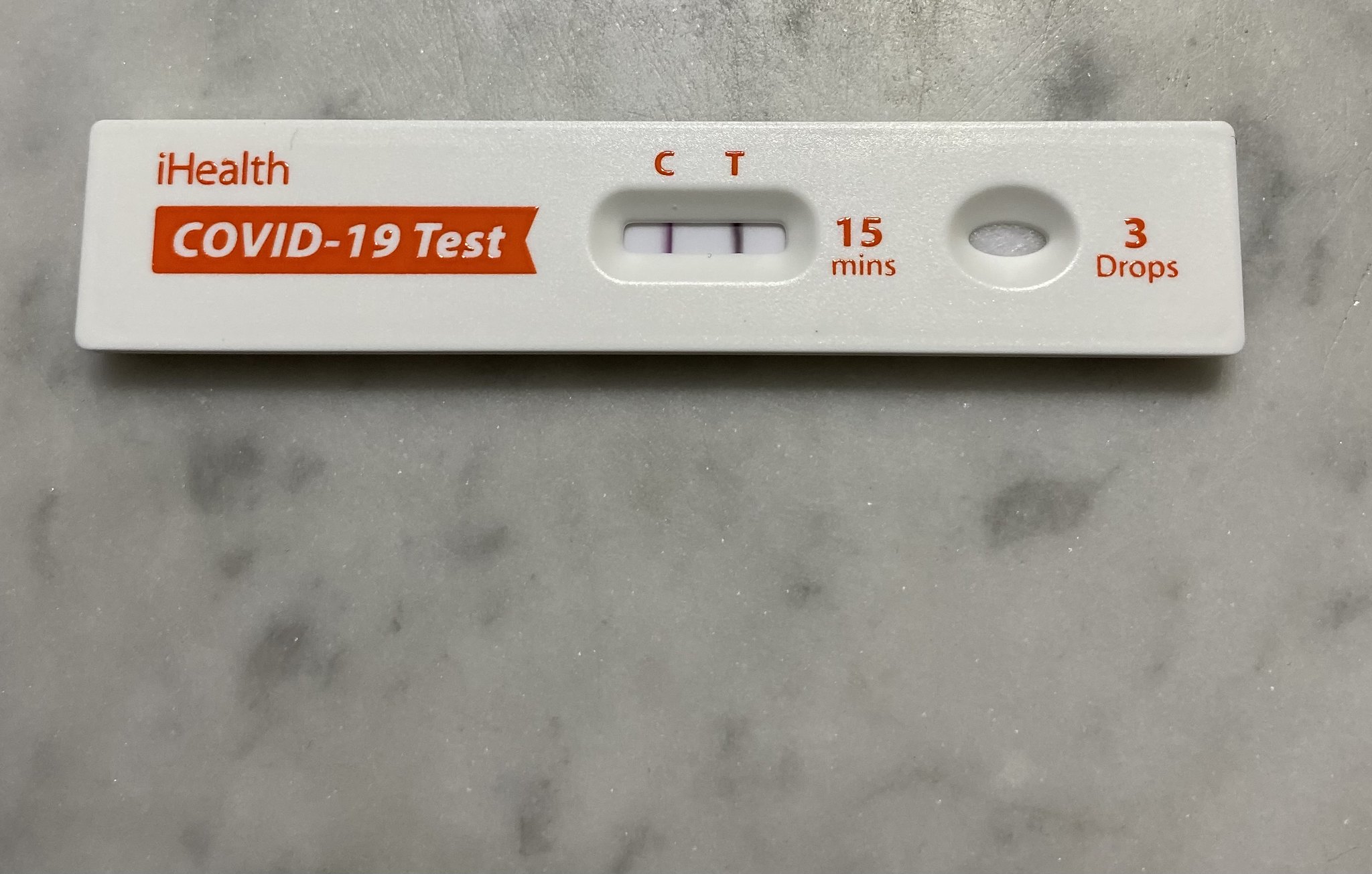The image features a splotchy, gray background with various shades of gray and occasional green-gray patches. Against this backdrop, a white, rounded rectangle stands prominently in the center. The rectangle displays the brand name "iHealth" in a somewhat orange-red hue. Beneath this, an orange-red banner with the text "COVID-19 Test" in white is visible. 

Towards the center of the rectangle, there are two key elements: an "C" and "T" printed in orange, accompanied by two horizontal black lines on a white background, suggesting test result indicators. Adjacent to this, the duration "15 MINS" is also printed in orange. 

Further down, a small circular dip encases an oval shape with a gray background. Next to this oval, the instruction "three drops" is indicated in red, with a faint black shadow falling beneath the text and icon, adding depth to the image.